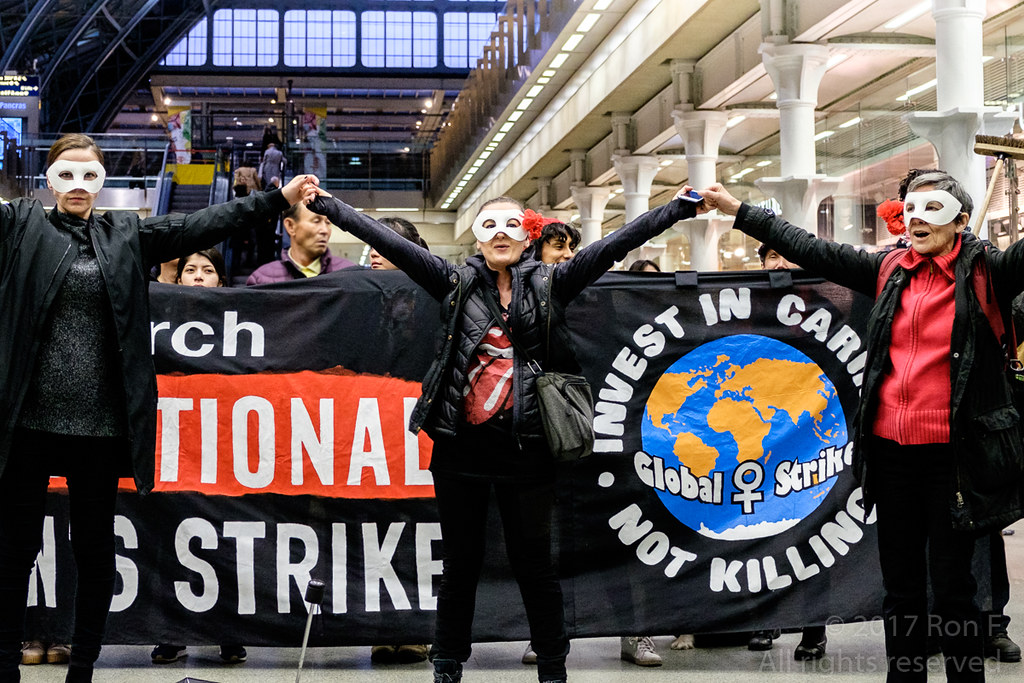This close-up image captures a group of protestors in what appears to be a large indoor public space, possibly a mall or train station, identifiable by the glass windows, white pillars, and visible escalators in the background. Three women stand in the foreground, each wearing black coats and pants with different colored shirts underneath. Their arms are raised and intertwined, and their faces are partially covered by white eye masks, reminiscent of Phantom of the Opera masks. Directly behind them, a large rectangular black banner stretches across the image, although portions of the text are obscured by the protestors. The banner features white lettering with a red section on the left, the partially visible letters "RHC" possibly indicating "national strike," and a graphic on the right. The graphic includes a globe with the words "Global Strike" and the phrase "Invest in Caring Not Killing" surrounding it. A transparent watermark in the bottom right corner states "Copyright 2017. All rights reserved."